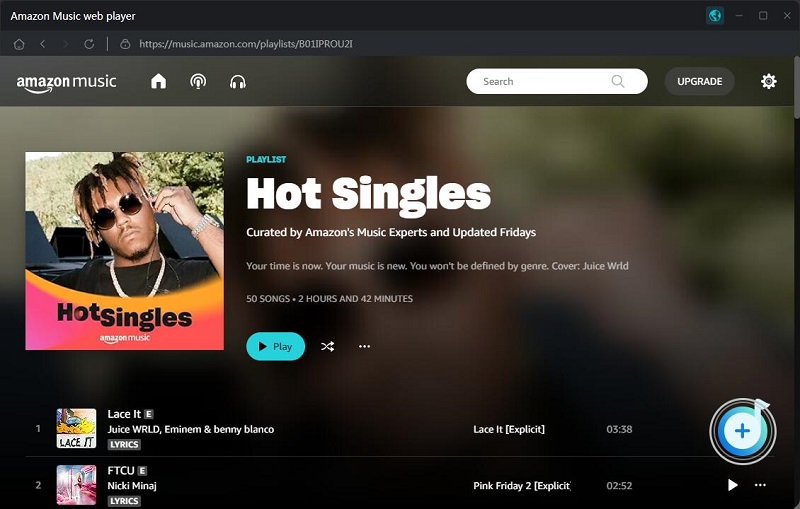This image is a detailed screenshot of the Amazon Music Web Player interface. In the upper left corner, the text "Amazon Music Web Player" is prominently displayed. On the opposite side, in the upper right corner, you can find an earth icon next to the minimize, maximize, and close buttons. Below the top bar, there's a navigation bar featuring a home button, back and forward navigation buttons, a reload button, and a web address bar displaying the URL "https://music.amazon.com/playlists/801PROU2I".

Just below this, the Amazon Music interface begins, with "Amazon Music" written in bold white letters. The navigation options here include a home button, an antenna icon, a microphone icon (mistakenly referred to as headphones), a search bar to the right, an upgrade button, and a settings gear icon.

Further down, the interface highlights a featured playlist section titled "Playlists, Hot Singles, curated by Amazon Music experts and updated Fridays." This section encourages users with the tagline "Your time is now, your music is new, you won't be defined by genre." Featured prominently is the "Hot Singles" playlist, showcasing a cover image of the late rap artist Juice WRLD. The playlist contains 50 songs with a total playtime of 2 hours and 42 minutes.

At the center, there's a green play button for immediate playback, a shuffle button, and a three-dot menu for more options. Accompanying the playlist are images and titles related to the featured artists and songs, including "Lace It" by Juice WRLD, Eminem, and Benny Blanco. The label "Hot Singles" and "Amazon Music" is reiterated next to the playlist cover.